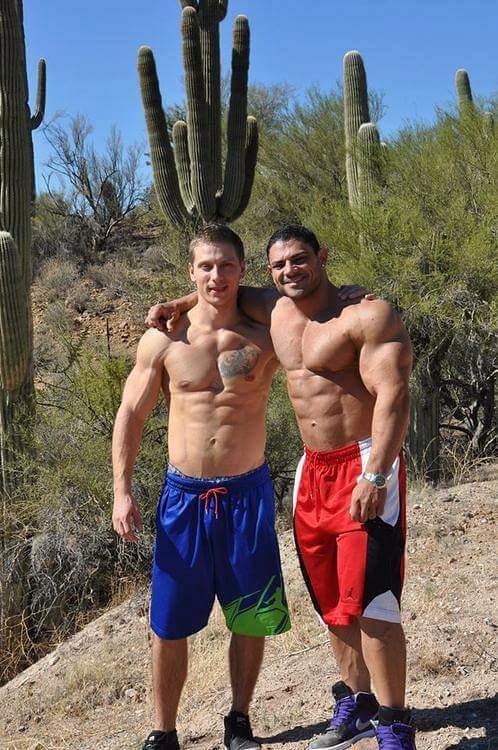The photograph depicts two very muscular, shirtless men standing in a desert landscape with several cacti and sparse vegetation, such as some dried grass and shrubs, set against a clear, blue sky. The man on the left, who is lighter-skinned and possibly Caucasian, has slightly smaller muscles and sports a tattoo on his chest. He is wearing blue shorts with an orange drawstring, a lime green accent on the bottom right leg, and black shoes. The man on the right has a tanner complexion and dark brown hair, suggesting he could be of Mediterranean or Hispanic descent. He is more muscular than his companion and is dressed in red shorts with white and black accents, black Nike shoes with purple laces, and an expensive-looking watch. The two men have their arms around each other’s shoulders, indicating a close bond as they pose confidently on a rocky, arid terrain.